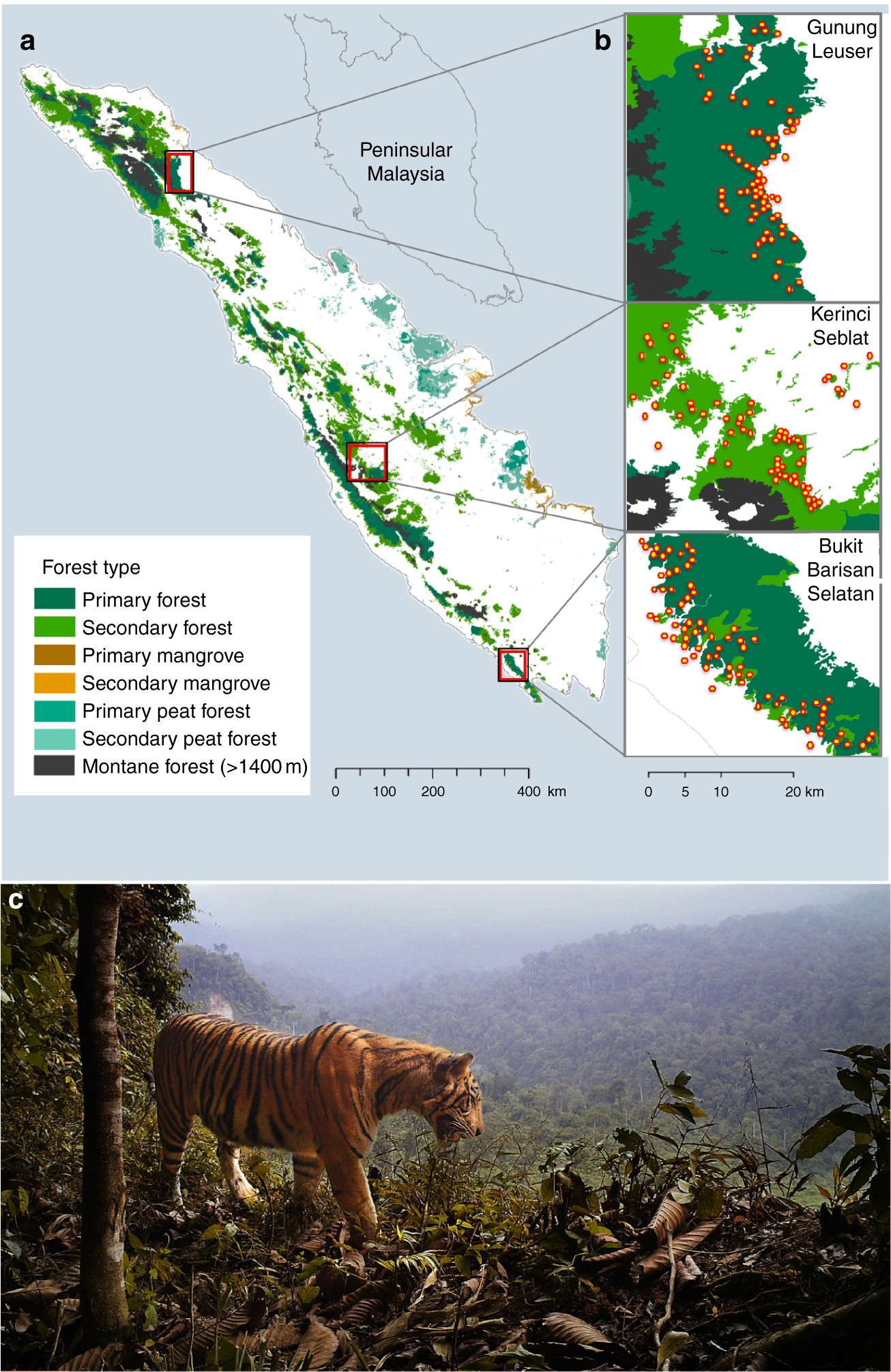This image consists of two parts. The upper section features a larger map, prominently displayed in the upper-left corner. The primary map is white with green regions, indicating areas of Peninsular Malaysia, a known habitat for Bengal tigers. In the upper-right corner, there is a green zoomed-in map of a region labeled "Ganag Luzur," which is a section highlighted on the main map to the left. This emphasized detail provides a closer look at a specific area within the larger geographic context.

Highlighted on the map are various locations marked with orange dots. Below the green map, additional regions are labeled as "Currency Sublot" and "Buket, Parisian, Sulayton." 

Below this cartographic section, the lower part of the image features a photograph of a Bengal tiger. The tiger is set within a forested environment, intently gazing at some leaves, perfectly illustrating the majestic creature in its natural habitat.